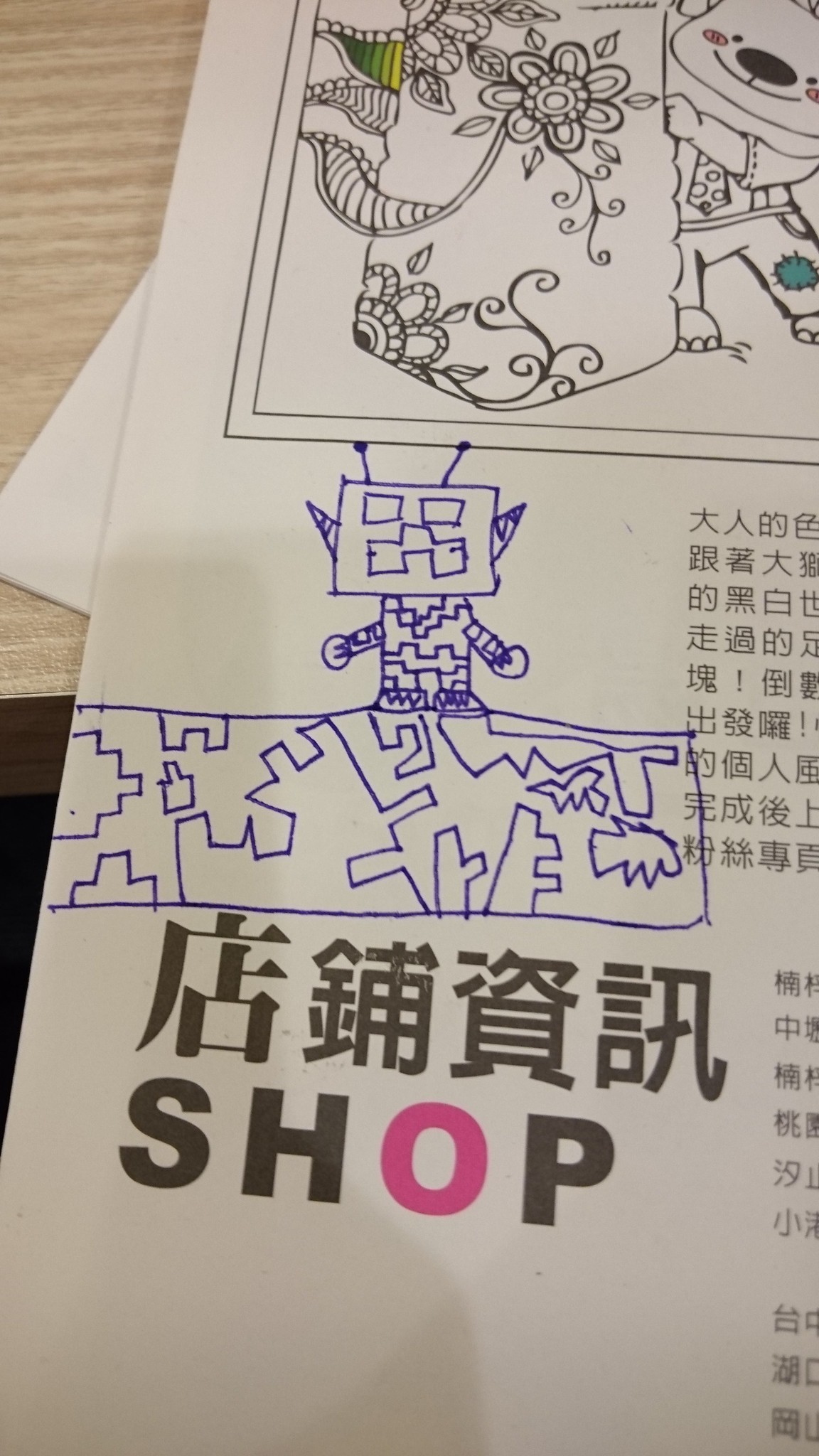The image features a sheet of paper, the exact nature of which is ambiguous - it could be a receipt, a pamphlet, or another type of document. The paper contains text in a foreign language, likely Japanese, and the only discernible English word is "SHOP" at the bottom, with all letters in black except for a pink "O." 

In the center of the paper, someone has drawn a small robot in blue pen. The robot is depicted standing on an assortment of shapes, which could be interpreted as rocks or similar objects. 

At the top of the paper, there is a printed image, unlike the hand-drawn robot. This printed section features flowers and vines, and a small animal, possibly a bear, holding the flowers. The overall layout and style suggest that this paper could be a page from a coloring book.